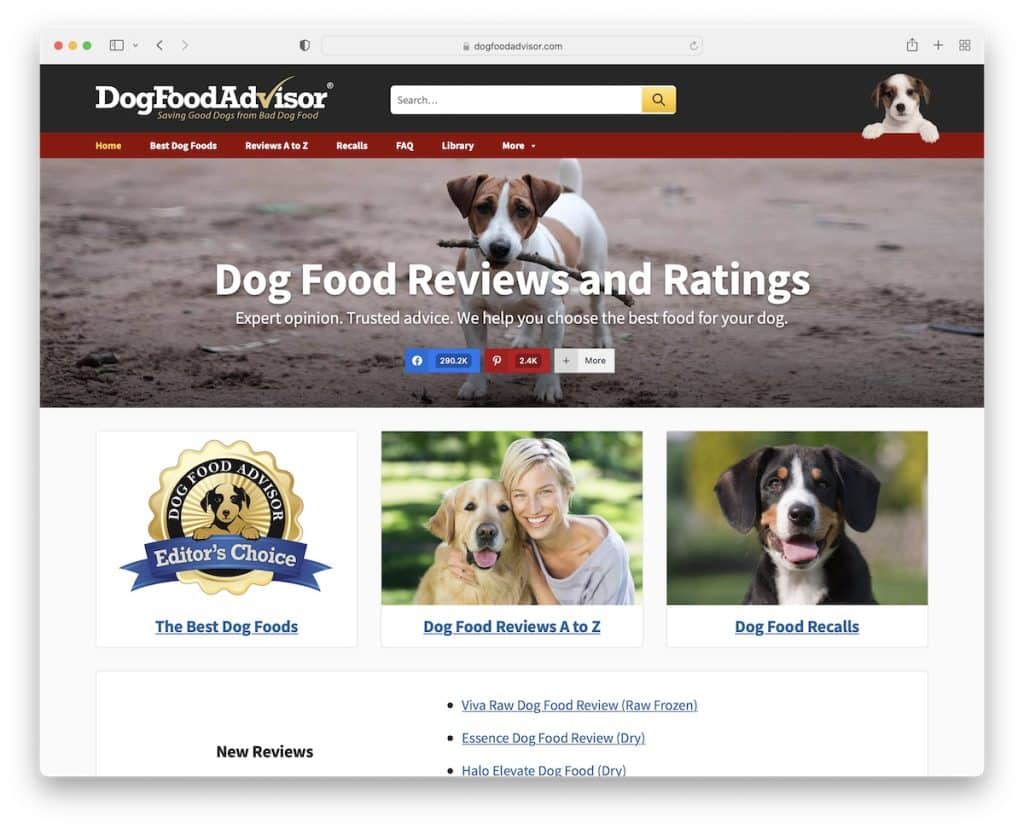This image, sourced from DogFoodAdvisor.com, exudes an inviting and informative atmosphere aimed at helping dog owners make informed choices about their pets’ nutrition. In the upper section, a search button is prominently displayed, encouraging users to explore the site’s offerings. To the right of the search bar, a charming brown and white puppy draws attention.

A series of headlines and subheadlines convey the website's purpose: providing dog food reviews and ratings, expert opinions, and trusted advice to aid users in selecting the best food for their pets. The site boasts an “Editor’s Choice” section and features the Dog Food Advisor logo, which links directly to a page highlighting the best dog foods available.

On the right, an image showcases a smiling woman beside her golden retriever, reinforcing the site's theme of nurturing canine companionship. Beneath this, a link directs users to comprehensive “Dog Food Reviews A to Z.” Further to the right, a healthy-looking black, white, and brown dog is pictured, accompanied by a link for dog food recalls.

Additional links guide visitors to detailed reviews, such as the “Viva Raw Dog Food Review” focusing on raw frozen options, and the “Essence Dog Food Review” covering dry food. This thoughtfully arranged layout assures users that they have everything they need to make the best dietary choices for their furry friends.